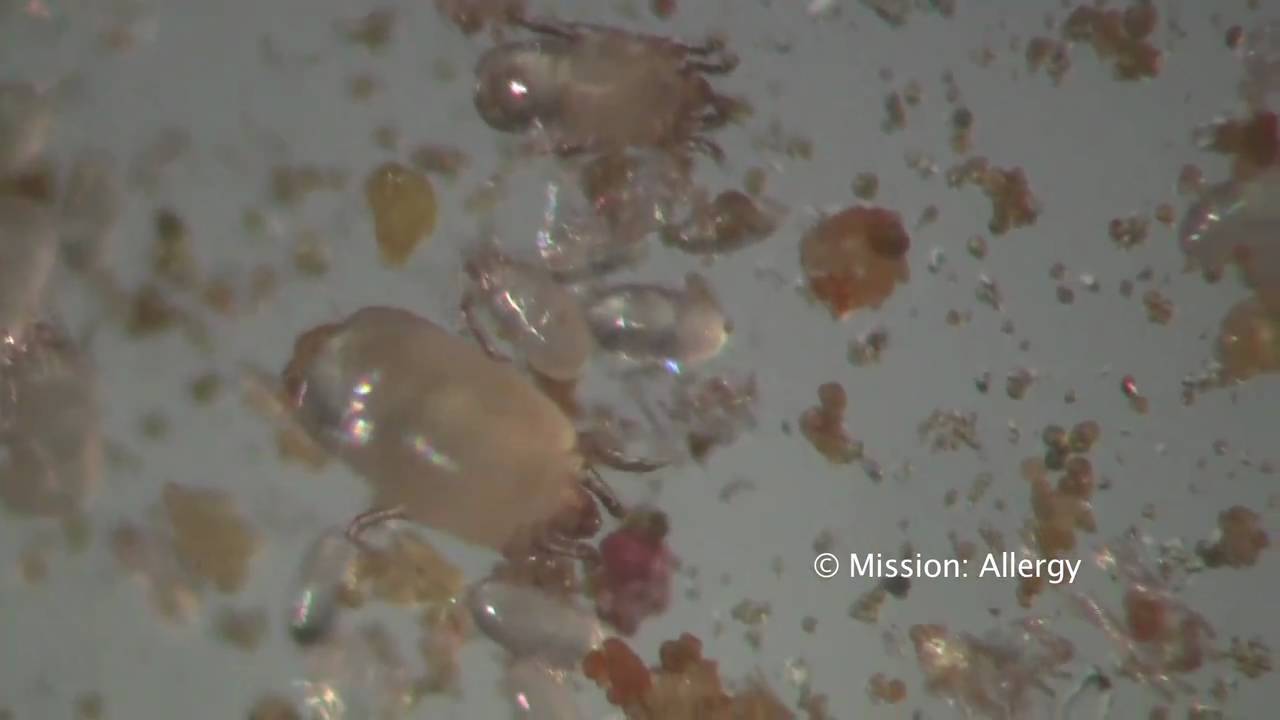This is an extreme close-up image of a dark gray, horizontally-oriented rectangle backdrop, overlaid with various splattered liquid textures. The splatters encompass a spectrum of browns—from light to dark—with some hints of greenish-brown. These fluid shapes form an eclectic mix of oval, circular, and dot-like formations, some with jagged edges. The sizes of these splatters range from minuscule dots to larger areas about the size of a fingertip. Additionally, there are transparent and orangish elements, adding to the visual complexity. Near the bottom right-hand corner, the text "mission... allergy" is clearly visible in white. The overall effect is reminiscent of randomly splattered gel or fluid on a dark surface.